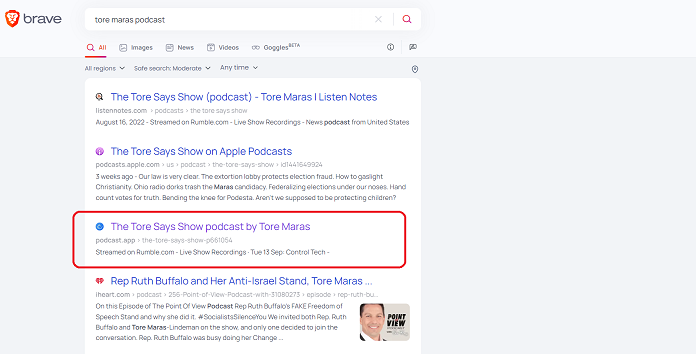This image showcases a webpage from the Brave browser, featuring a search result page. The focal point of the screen is a search bar adjacent to the Brave logo. Beneath the search bar, the query "Tora Mara's podcast" is shown. The results that appear are highlighted in orange, indicating they are selected or prioritized.

The first result displayed is titled "The Tori Says Show Podcast with Tori Maras," from the platform Listen Notes. 

Next, two results are listed under "The Tori Says Show." One result is from Apple Podcasts, including a brief description within an outlined red box. It reads: "The Tori Says Show Podcast by Tora Maras," featuring a small blue icon next to it.

The final piece of information concerns a specific episode titled "Representative Ruth Buffalo and Her Anti-Israel Stand," from the podcast "The Point of View." The description mentions Representative Ruth Buffalo's so-called "fake freedom of speech standard" and discusses the reasons behind it. This suggests that the podcast does not shy away from addressing controversial subjects, indicating a bold approach to covering a range of topics.